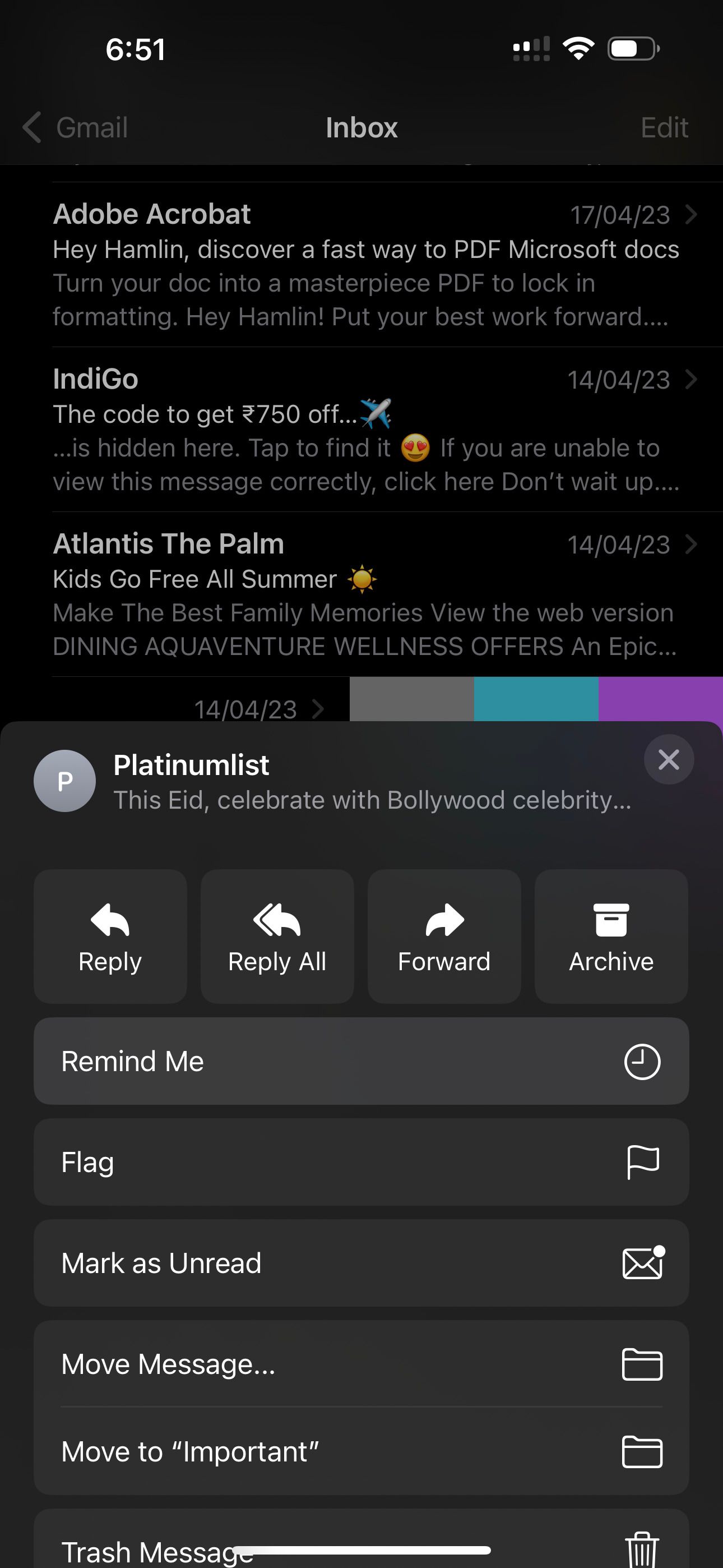This image is a screenshot captured from a cell phone, illustrating the user's Gmail inbox. The background appears to be very dark, which highlights the white text prominently displayed in the foreground.

In the upper left corner, the time 6:51 can be seen, while the top right corner shows a battery level indicator at 60%. Centered at the top of the screen, the title "Inbox" is visible, with "Gmail" labeled to its left and "Edit" to its right.

The first email in the inbox is from Adobe Acrobat, carrying the subject "Hey, Hamlin, discover a fast way to PDF Microsoft Docs," indicating a promotional email. The second email is from Indigo, with a subject line reading "The code to get $7.50 off," accompanied by a small avatar, suggesting another promotional or spam message. The third visible email is from Atlantis The Palm, with the subject "Kids go free all summer," which also appears to be promotional in nature.

At the bottom of the screenshot, the app drawer or options menu from the email app is open. It lists various actions for the selected email, including "Reply," "Reply all," "Forward," and "Archive." Additional options available are "Remind me," "Flag," "Mark as unread," "Move message," "Move to important," and "Trash message." The text "Platinum List, this Eid, celebrate with Bollywood celebrity" appears just above the options, though its relevance to the email content is unclear.